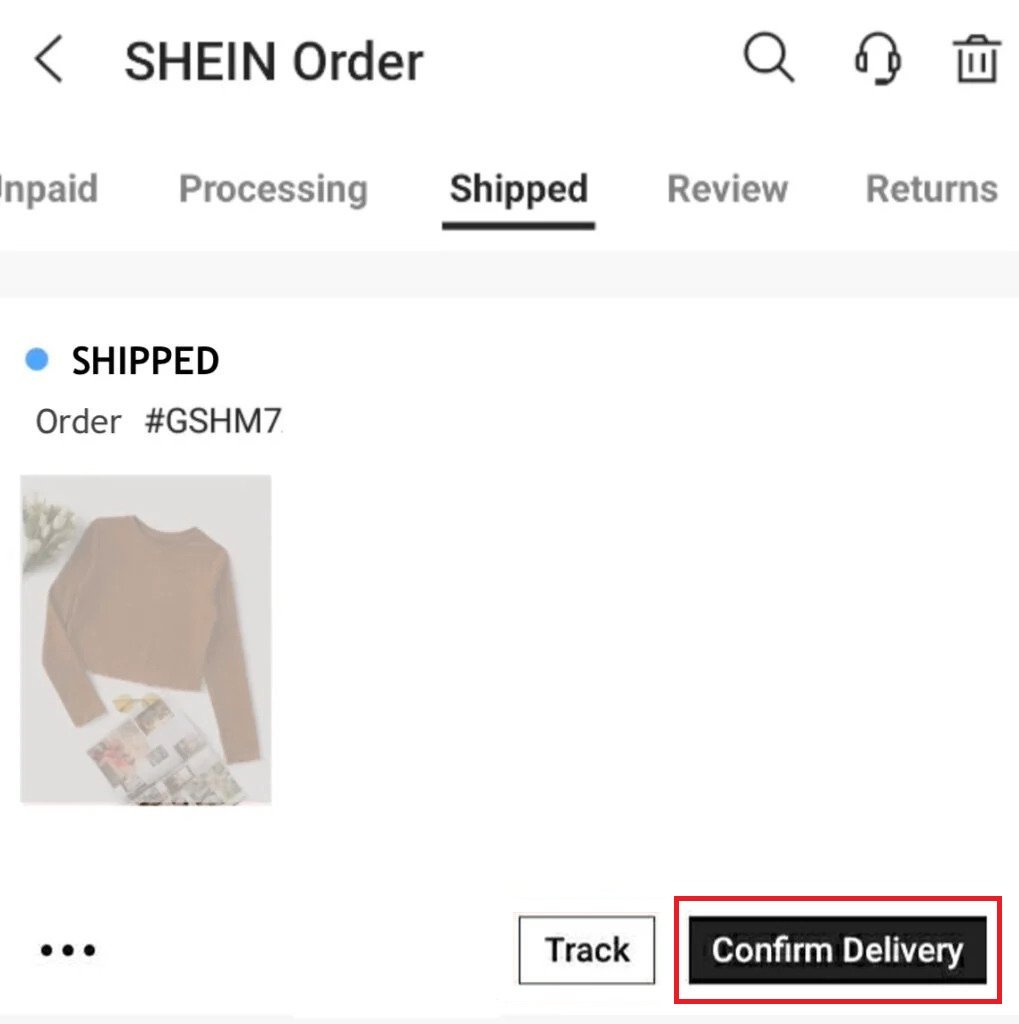The image depicts a section of a website, specifically an order tracking page from the Shein platform. 

- **Top Left Corner**: A light arrow is displayed, followed by the text "SHEIN" in capital letters, and "Order".
- **Icons**: Adjacent to the text, there is a magnifying glass icon (suggesting search functionality), a headphones icon (likely indicating customer support), a headset icon, and a trash can icon. 
- **Order Processing Details**: The page includes terms such as "Processing," "Shift," "View," and "Returns." The word "Shift" is bolded and underlined in black.
- **Miscellaneous Icons/Texts**: A blue circle is present, along with the order number "GSHM7".
- **Product Information**: Below this, there's an image depicting a shirt and a skirt with ellipses ("...") suggesting further information or a list.
- **Action Buttons**: 
  - A square button labeled "Track".
  - A rectangular button with a red border that reads "Confirm Delivery".
- **Bottom Right Corner**: The rectangle at the very bottom right is blacked out with a hint of a red border.

Overall, this seems to be a detailed view of a section for tracking orders on the Shein website, emphasizing the various elements and navigation options available to users.